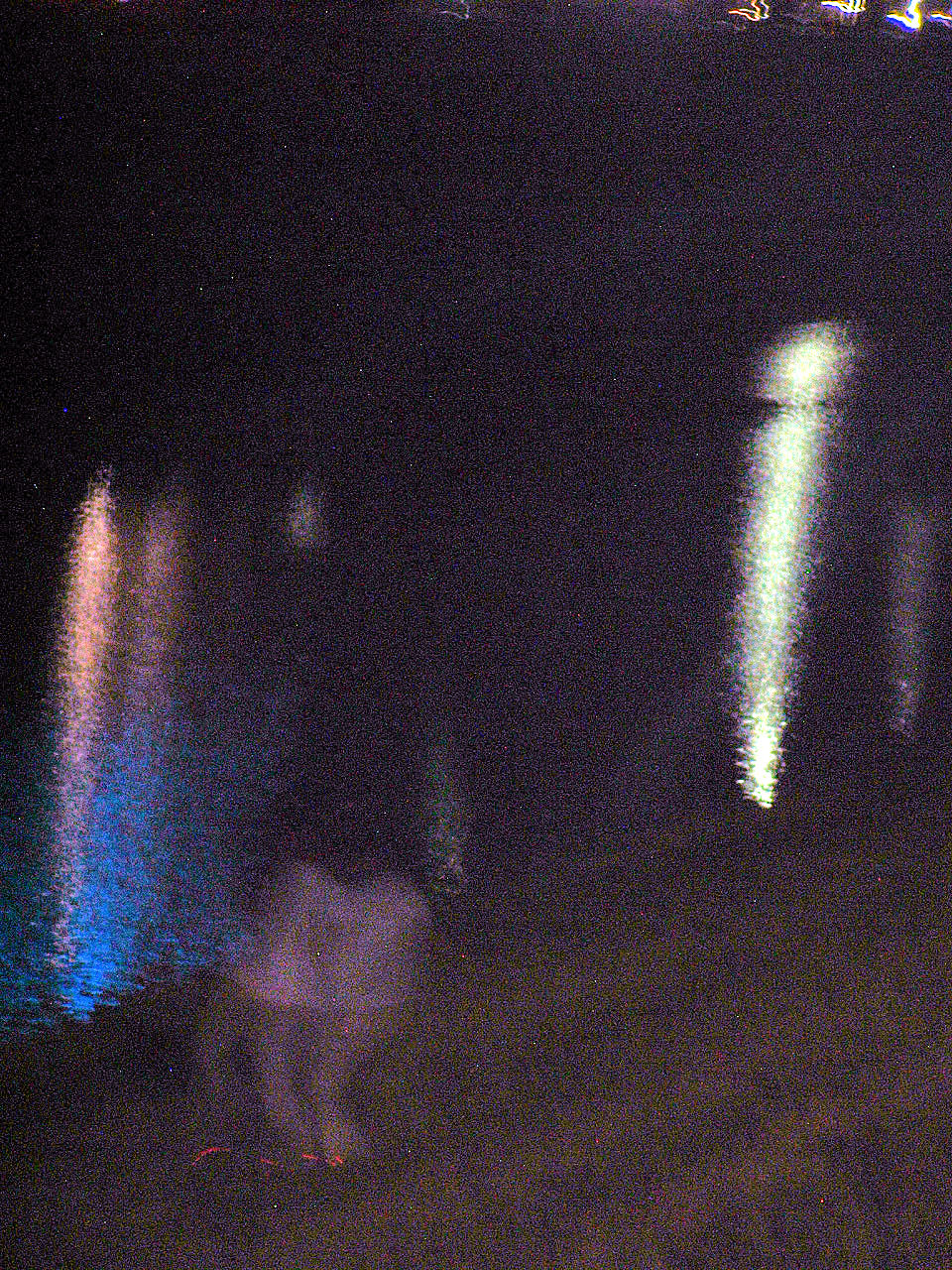This extremely blurry and distorted nighttime photograph appears to depict one or two people standing or walking near a body of water. The image is characterized by its low resolution and graininess, making it difficult to identify specific details. The background is predominantly dark, with areas of black and gray. There is a noticeable blue reflection on the water, which is cast by various lights present in the image. One prominent light, which is tall and white-yellow, is located on the right side, shining onto the water and creating a bright blur. 

Toward the bottom right corner, there is a gray triangular area, and moving towards the center-left, there appears to be a pinkish circle with three gray legs and four small orange dots, possibly indicating reflections or artifacts from the camera distortion. The potential figures seem to be wearing similar clothing, such as black shirts with possibly white sleeves and pink shorts or skirts. Near their feet, bright orange spots are visible, which could be painted toenails or objects on the ground.

Further details include two white stripes with a blue base on the left and a long blue stripe with a white dot at the top on the far right. Additional lights and faint squiggles at the top suggest a distant city or ambient lighting. Overall, the scene appears to be a water's edge, possibly a riverbank or beach, illuminated by various light sources on a dark night.